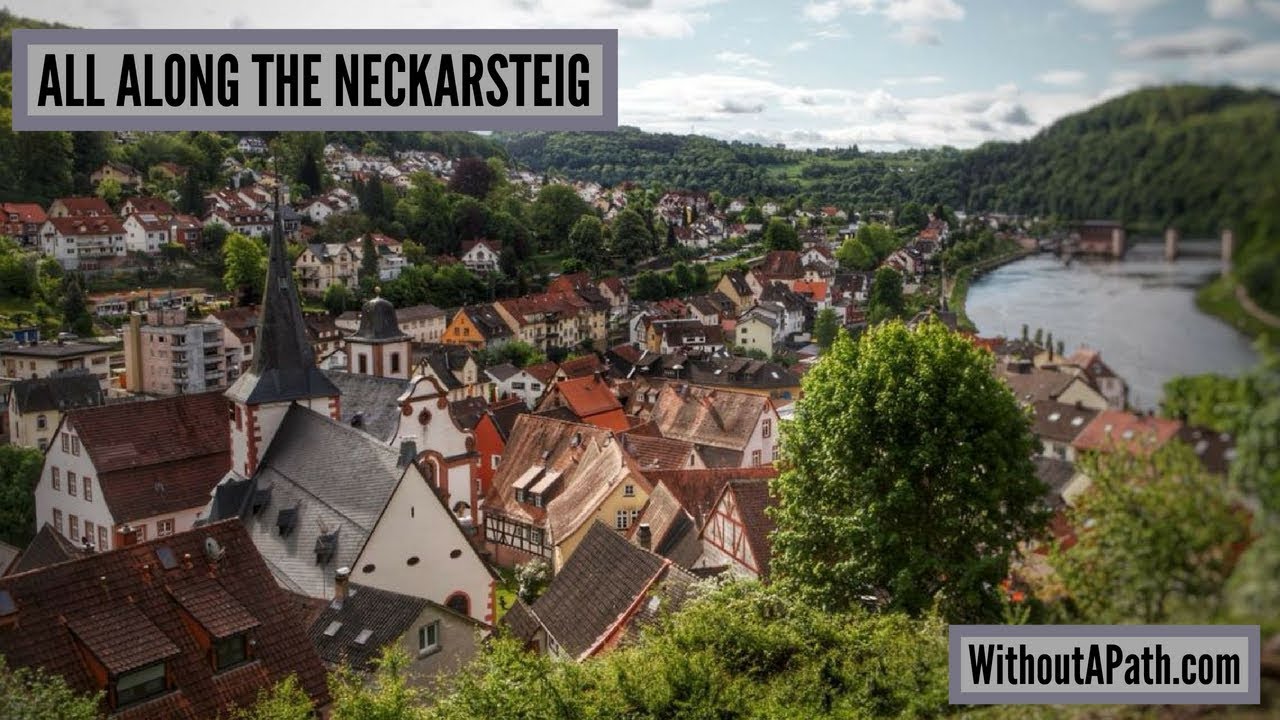This aerial drone shot, likely taken from atop a building or a hill, offers a detailed top-down view of a compact, traditional European town, possibly German, Swiss, or Austrian. The buildings, showcasing a variety of roof styles including heap, gable, mansard, and pitch roofs, appear centuries-old, enhancing the historical charm of the village. At the center stands a church, majestically surrounded by these quaint structures. The backdrop unfolds into lush green hills and imposing mountains, with a serene river gracing the right side of the image. The sky, a mix of clouds and scattered sunshine, adds a hint of coldness to the scene. Prominent texts adorn the image indicating, in the top-left corner, "all along the Neckarssteig," likely the town's name, and in the bottom-right corner, a watermark that reads "withoutapath.com," suggesting a travel blog or website. The predominant colors in the picture include various shades of blue, green, brown, gray, and yellow, enhancing the overall picturesque quality of the town.